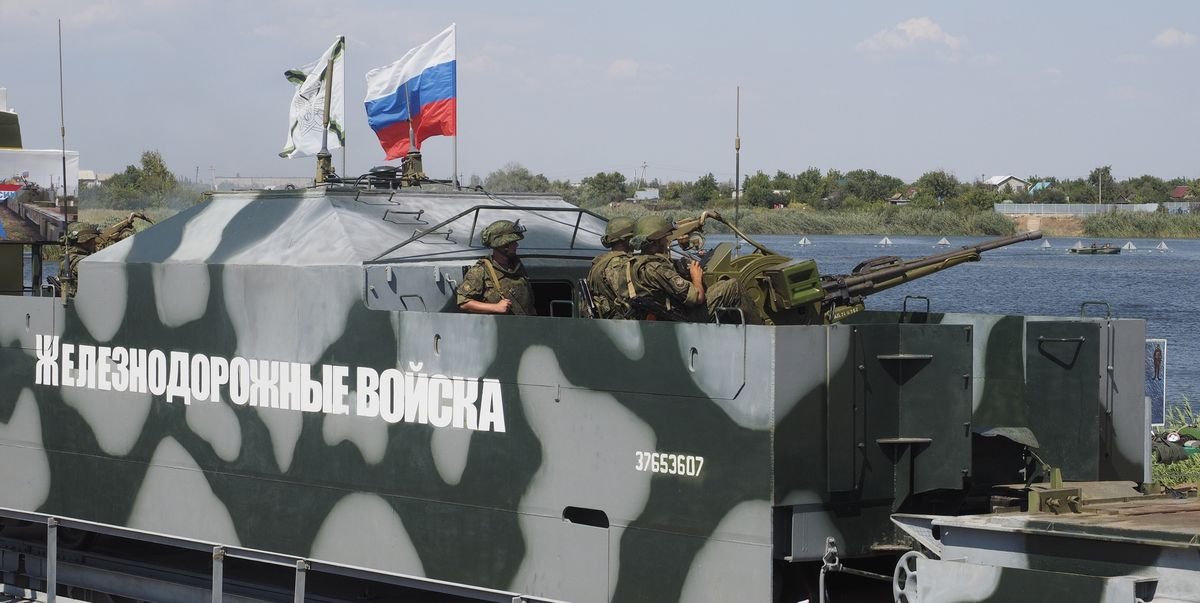The landscape-oriented color photograph features a Russian armored train, painted in dark green with gray camouflage patterns, that extends from the left side of the image to the bottom right. Near the head of the train, the number "3765-3607" is visible. Foreign text in Russian is inscribed on its side. On the upper portion of the central deck, two flags are flying: the Russian Federation flag with its horizontal stripes of white, blue, and red, and another white flag adorned with black and brown patterns. In the foreground, there are four soldiers in green camouflage uniforms and hats. One soldier is facing slightly downwards toward the viewer, while the others face the right side of the image, manning a long-range rifle. The scene is set near a body of water, with additional sailing vessels and buildings visible on the horizon. The photograph captures the detailed and realistic representation of the military scene.